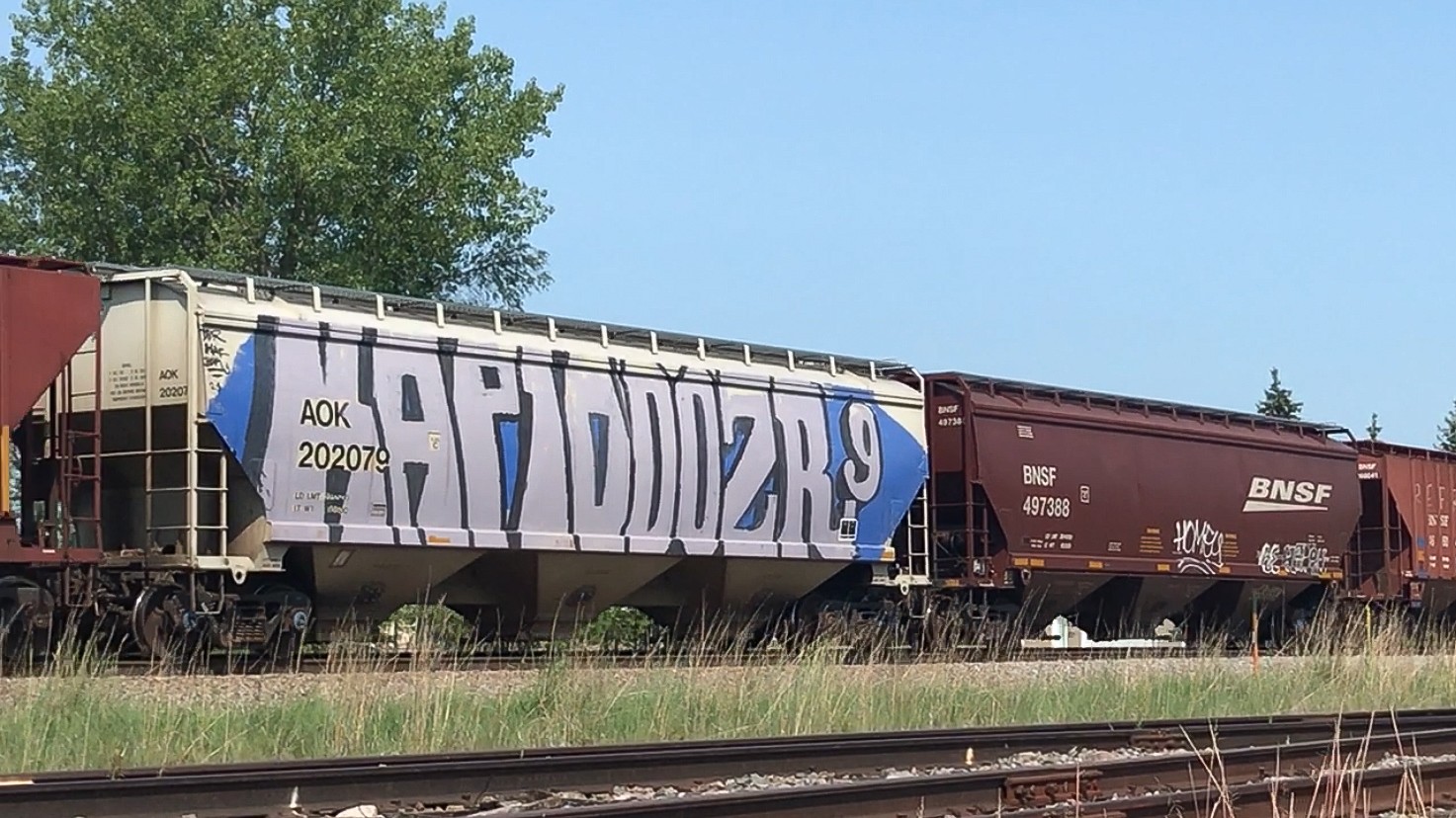The photograph captures a lineup of train cars parked on a track with a vivid natural backdrop. Dominating the left side, a white train car is adorned with elaborate graffiti featuring a blue background and striking white letters that seem to spell "KAP1000ZR" followed by a small "9". Above this colorful design, the pre-printed identifier "AOK202079" is clearly visible in black lettering. Adjacent to this, a brown train car stands prominently, marked by the large, black lettering "BNSF" on the right, and "BNSF497368" on the left. This car also has subtle white graffiti tags near its base. Further right, another reddish-brown train car is partly visible at the extremes of the frame. The bottom of the image reveals an additional set of tracks bordered by overgrown, wispy green weeds that add a lively touch to the scene. The vibrant greenery continues behind the train, crowned by a towering, lush tree set against a cloudless blue sky, enhancing the natural beauty surrounding the industrial elements.